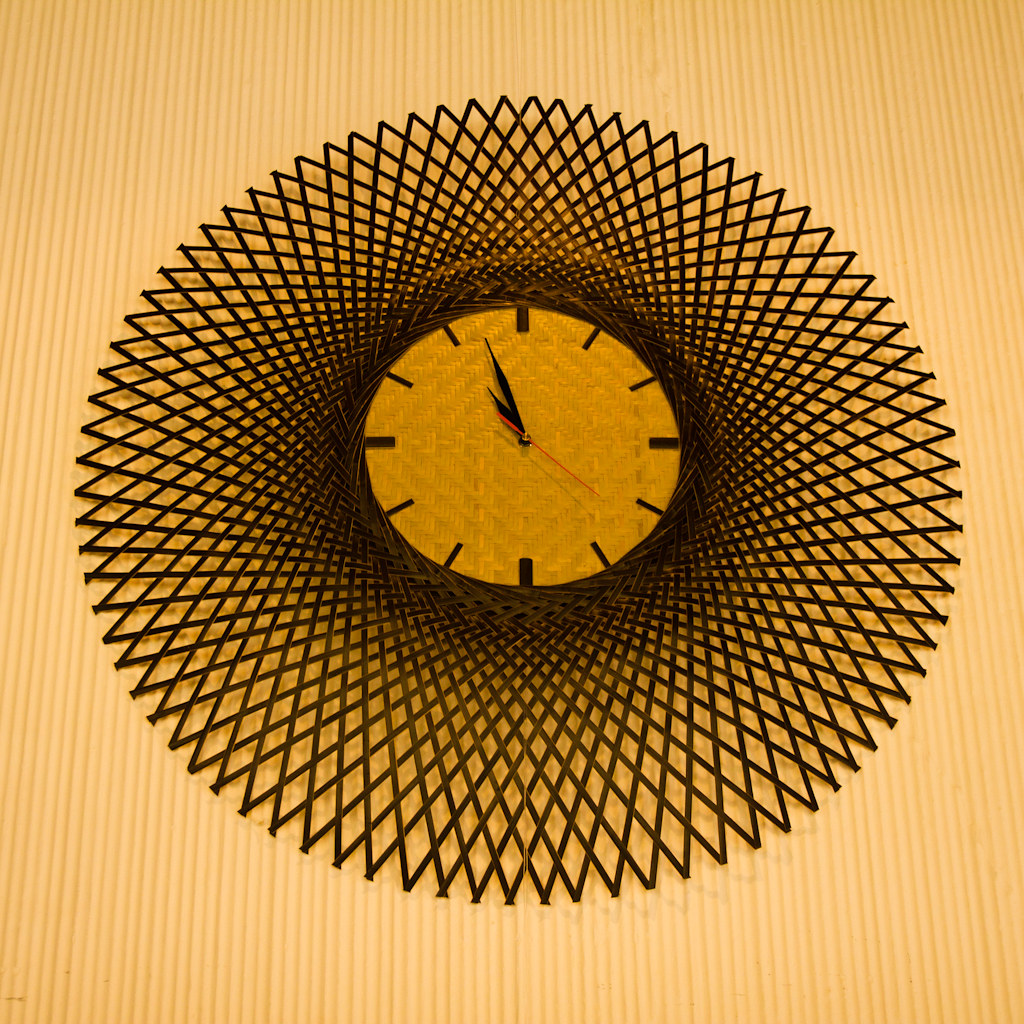This photograph features a striking wall clock set against a tan, bamboo-like background. The clock is adorned with an intricate crisscross pattern reminiscent of designs created with a spirograph, forming a lattice of diamond shapes that extend widely beyond the clock's face. The clock itself has a sophisticated tan or gold face, accented by sleek black hour and minute hands. The minimalist design eschews traditional numbers in favor of clean, black lines to mark the hours, while a vivid red second hand adds a touch of contrast. The time displayed is approximately three minutes to 11 o'clock.